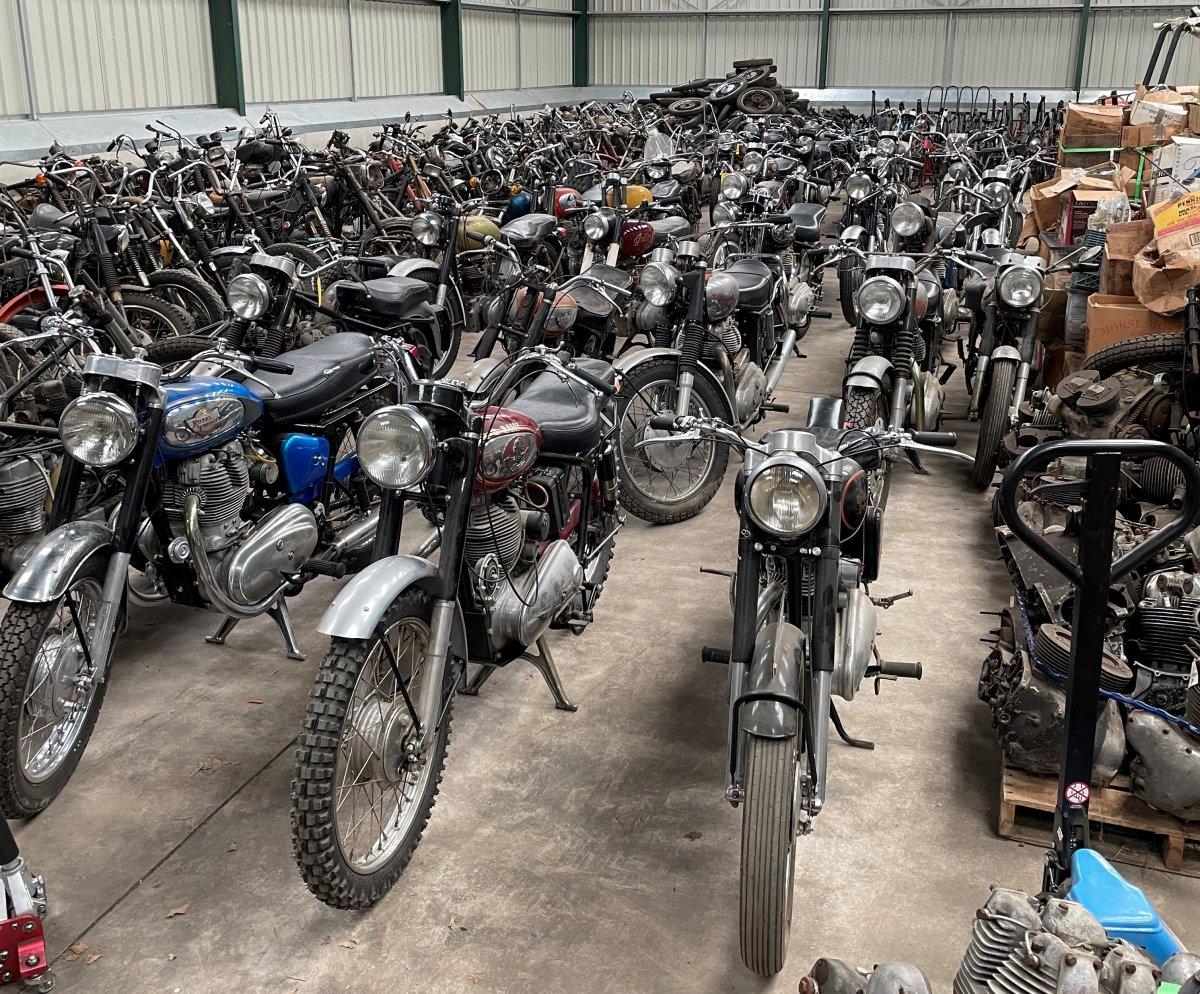The image depicts a vast indoor garage or shop with a gray concrete floor, lined with hundreds of vintage motorcycles. Each motorcycle features light gray metal fenders covering their black tires, and all are parked in neat rows. None of the headlights are illuminated. The motorcycles in the foreground face forward, while those on the left side are pointed to the right. In the upper right corner, there are cardboard boxes stacked, and nearby, there appears to be a device for carrying heavy equipment. The garage wall is constructed with vertical metal slats. Additionally, a pile of tires can be seen at the back of the shop along with what looks like engines and carburetors on the right-hand side. The setting is indicative of either a large private collection or a storage area for motorcycles, emphasizing the sheer number and vintage nature of these bikes.